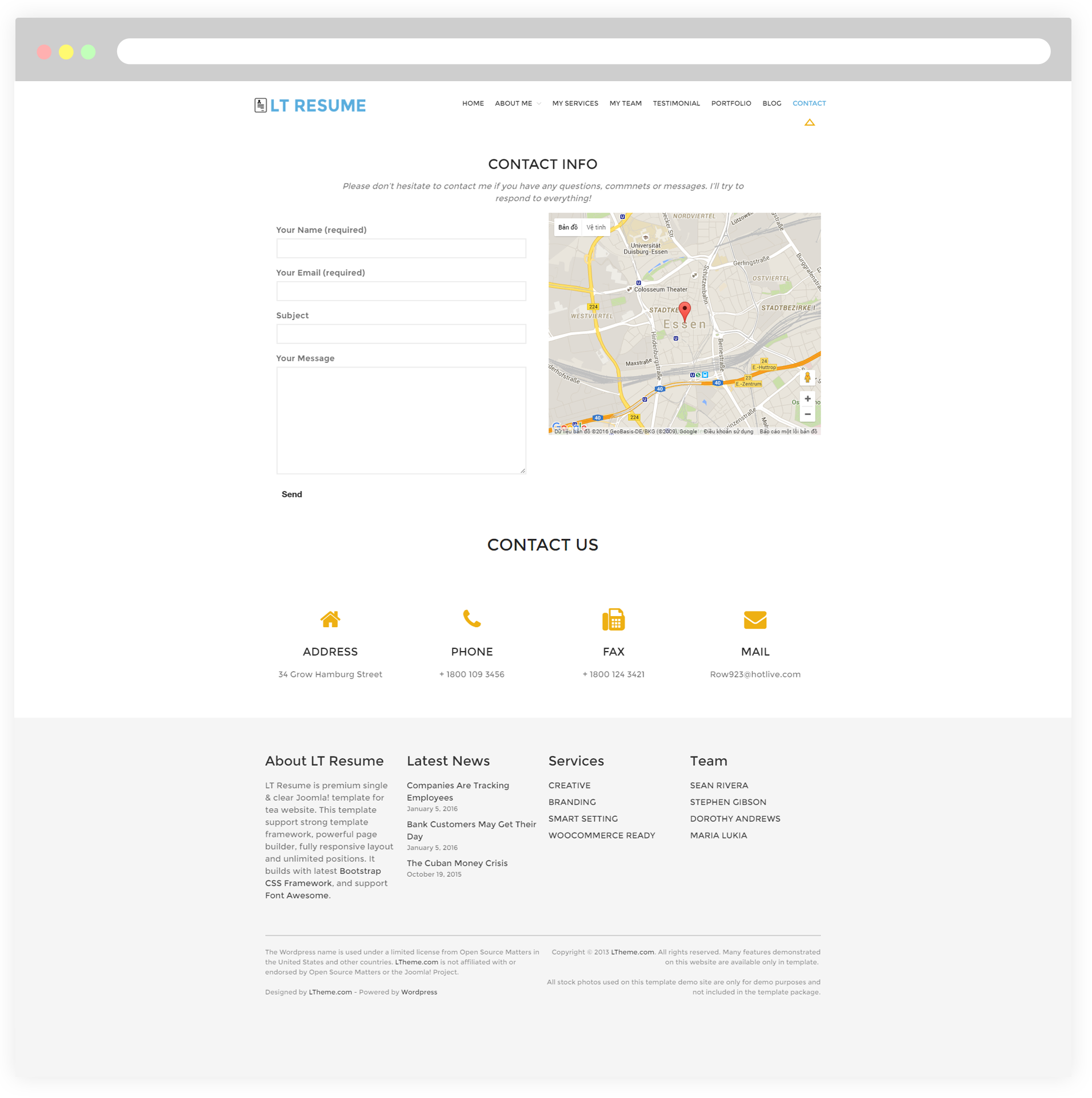The image features a web page layout with distinct sections and a well-organized design. At the very top of the page, there is a gray bar spanning the entire width. Inside this gray bar is a white search bar stretching from the left edge to the right. Positioned in front of the search bar on the left are three colored circles: red, yellow, and blue.

Below this horizontal bar, on the left side, there is bold blue text in all capitals reading "LT" followed by the word "Resume." To the right of this, a menu is displayed, consisting of seven selectable options, followed by an eighth option that is highlighted in blue. 

Centered below the menu is the heading "Contact Info," with two lines of text directly underneath it. To the left of this section is a list of four words, while on the right side, there is an illustrated map. The map depicts yellow roads and features a red location marker.

Beneath the map, centered, the words "Contact Us" are prominently displayed, followed by a dividing line. Under this line, there are icons in orange: a house representing the address, a phone symbolizing the phone number, a fax machine icon, and an envelope for email.

At the bottom of the page, there are four columns. The first column is labeled "About LT Resume," the second "Latest News," the third "Services," and the fourth "Team."